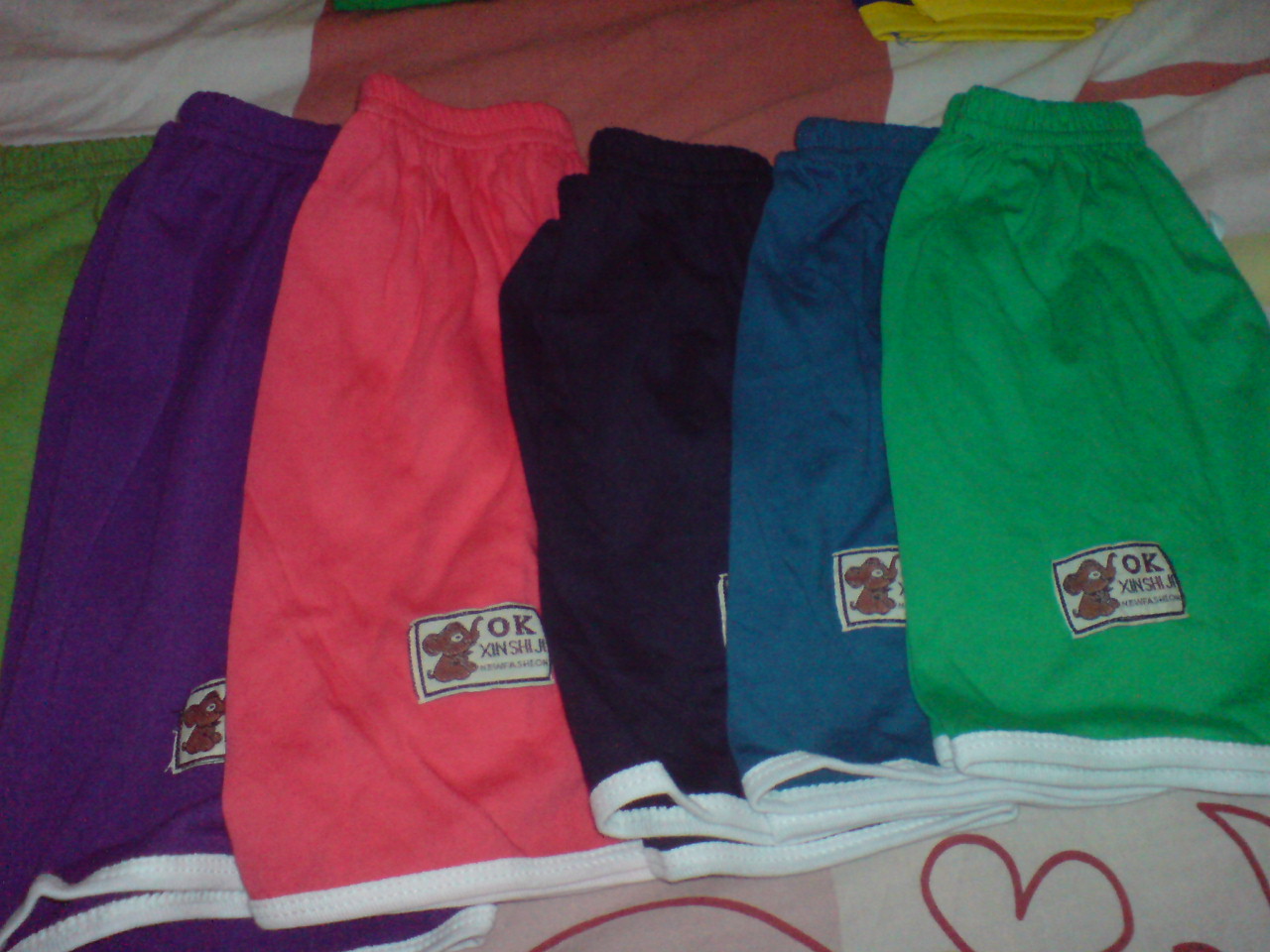The image depicts a lineup of five pairs of children's athletic shorts, each uniquely colored, ranging from dark green to vibrant purple, pinkish-red, black, and a grayish royal blue. They are folded in half and laid atop each other, fanning out horizontally across a white, pink, and light red patterned fabric background. Each pair features an elasticated waistband and has a white contrast trim around the leg openings. A small fabric tag, stitched onto the front of the right leg, displays a dark brown elephant silhouette and the letters "OK" in brown text on a white background, denoting the brand. The overall presentation is a close-up, showcasing the details and colors of the shorts distinctively.